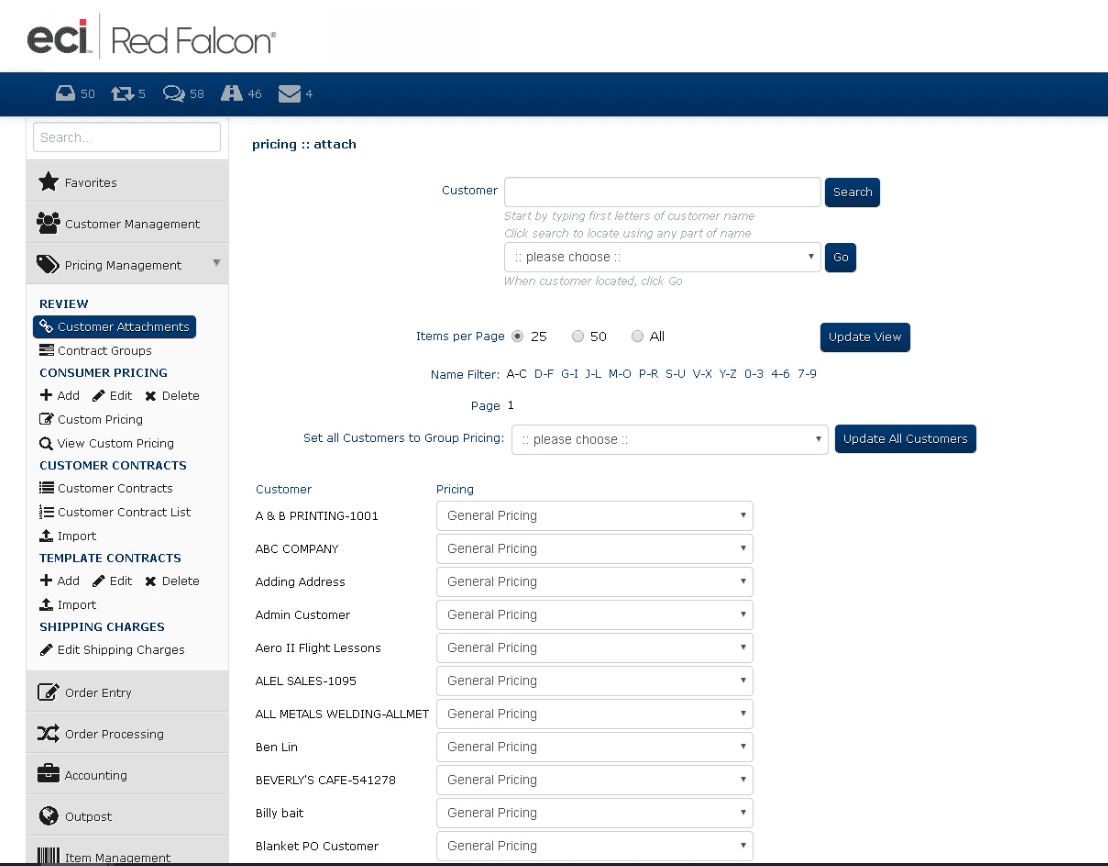The image depicts a detailed web page interface for a platform labeled "SECECI". The word "SECECI" is prominently displayed in black letters at the top of the page, with a red square dotting the "I". A line extends right from the "I" to the label "Red Falcon."

Directly beneath this header, a blue navigation bar runs across the width of the screen, featuring several icons and numerical notifications in white. Starting from the left, there's an inbox icon resembling a box with the number "50" beside it. Next to that, a set of looped arrows indicates a sync or refresh function, with the number "5" below it. Following this are word balloons representing a messaging function marked with "58". To the right, an icon of a roadway is accompanied by the number "46", and lastly, an envelope icon with the number "4" completes the notification section.

The web page is divided into two main sections. The left side features a vertical navigation panel that includes numerous menu options such as "Favorites," "Customer Management," "Pricing Management," "Order Entry," "Order Processing," and more. Additional options in this panel include "Template Contracts," "Shipping Charges," "Customer Contracts," and "Consumer Pricing Selections."

Taking up the majority of the right side is a workspace area labeled "Pricing Attach." This section contains a series of boxes designed for customer interaction. At the top of this area is a customer search box, followed by a name filter that organizes letters of the alphabet and numbers 1-9 into three-character groups, allowing users to filter names that start with a selected character.

Below the filters, there is a list of customers that includes businesses such as "A and B Printing" and "ABC Company," ending with "Blanket PO Customer." Each customer entry is accompanied by an empty box labeled "General Pricing," which includes a down arrow icon suggesting that the user can expand the box to make more detailed selections.

This detailed breakdown highlights the comprehensive functionality and user interface elements designed to facilitate customer and pricing management operations on the platform.